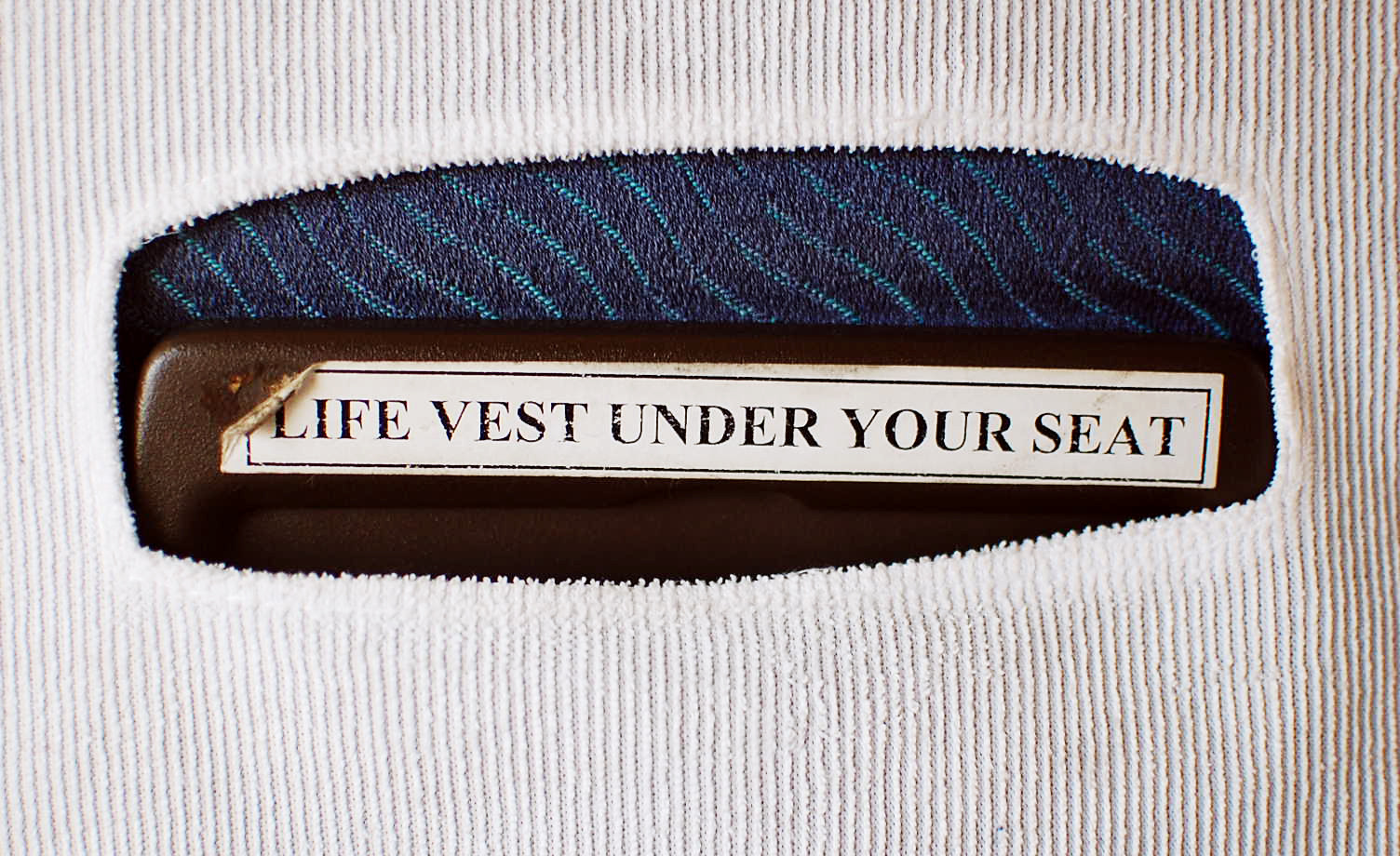The image depicts a textured, white fabric platform resembling a cushion or upholstered surface, with vertical brown lines running across it. In the center of the platform, there is a rectangular cutout featuring a blue and purple material with diagonal blue lines. Below this material, a white label with black borders, slightly peeling at the top left corner, bears the text "LIFE VEST UNDER YOUR SEAT" in all caps. The label is attached to a brown leather-like platform. The contrasting textures and colors, including the ribbed white fabric and the smooth blue and brown materials, create a visually engaging composition focused on the safety message.